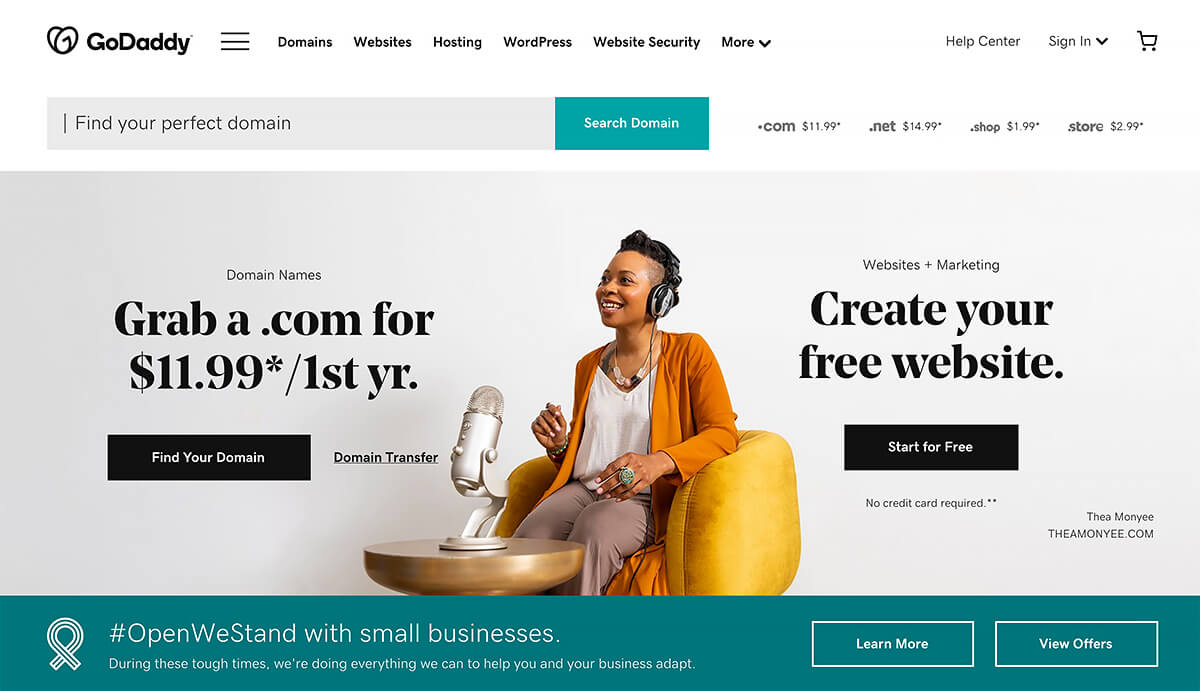This screenshot captures the homepage of the GoDaddy website. At the top of the page, there is a white navigation bar featuring a small heart-shaped icon next to the "GoDaddy" logo in black font. Adjacent to this logo are three horizontal lines indicating a menu, followed by the navigation options: "Domains," "Websites," "Hosting," "WordPress," "Website Security," and an "More" dropdown menu indicated with a small downward arrow. Further along the navigation bar are links to the "Help Center," "Sign In" option with an additional dropdown arrow, and a shopping cart icon.

Directly below the navigation bar is a grey search field labeled "Find Your Perfect Domain," accompanied by a teal "Search Domain" button in white font. To the right of this search section, a listing of domain pricing is displayed in red font: ".com, $11.99," ".net, $14.99," ".shop, $1.99," and ".store, $2.99."

The main content area of the webpage is dominated by a large grey rectangle. At the center of this area is a prominent photograph of a woman of African descent. She has short, black hair that is shaved on the sides and is sitting in a bright yellow, puffy chair. The woman is oriented towards the left, smiling, and wearing headphones, adding a personal and engaging visual appeal to the website.